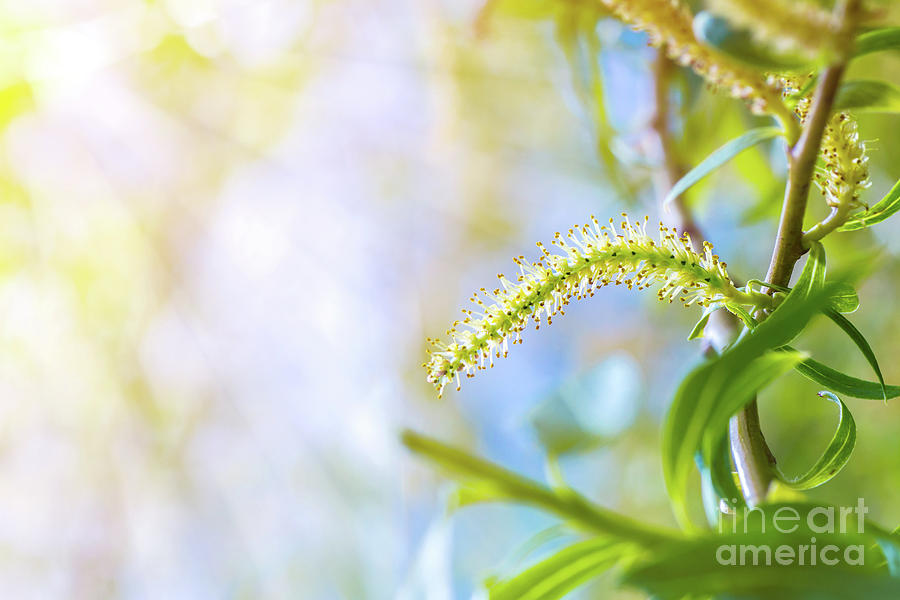This finely detailed close-up photograph, presented in landscape style, showcases a vivid green plant bathed in sunlight. The plant's brownish stem supports a stalk adorned with dozens of thin, white, hair-like protuberances—each capped with tiny green dots—giving it an almost caterpillar-like appearance. The vibrant leaves are green and thin, contributing to the lush, colorful palette of the image that includes greens, yellows, and touches of brown. The sunlight beams down from the left, casting a soft, muted glow that blurs the background, making the intricate details of the plant stand out prominently. In the bottom right-hand corner, the label "Fine Art America" signifies the photograph's high-quality artistry.